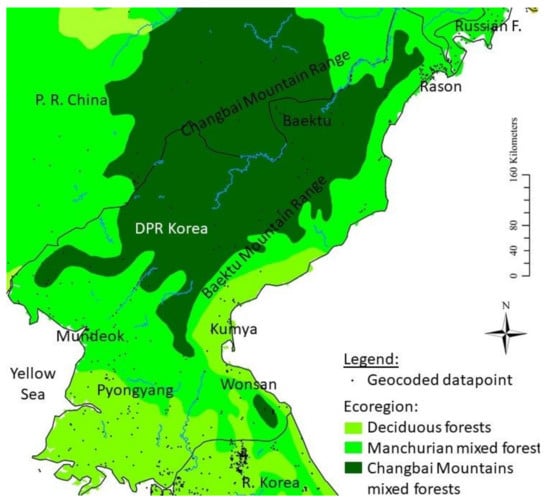This detailed geological map highlights various eco-regions across parts of North Korea (DPR Korea), China (PR China), and Russia. The landmasses are depicted in varying shades of green to indicate different forest types: light green for deciduous forests, medium green for Manchurian mixed forests, and dark green for Changbai mountains mixed forests. The map also features numerous labeled regions in black or white text, including "DPR KOREA," "PR CHINA," and "RUSSIA," among others. The background of the map is white, offering clear contrast to the colored regions. A legend in the bottom right corner clarifies the color meanings and includes geocoded data points. Additionally, a scale and a compass for directional reference are located on the right side of the map. The map covers a significant part of North Korea towards the bottom, China in the top left, and Russia in the top right, providing a comprehensive view of the forested areas within these countries.